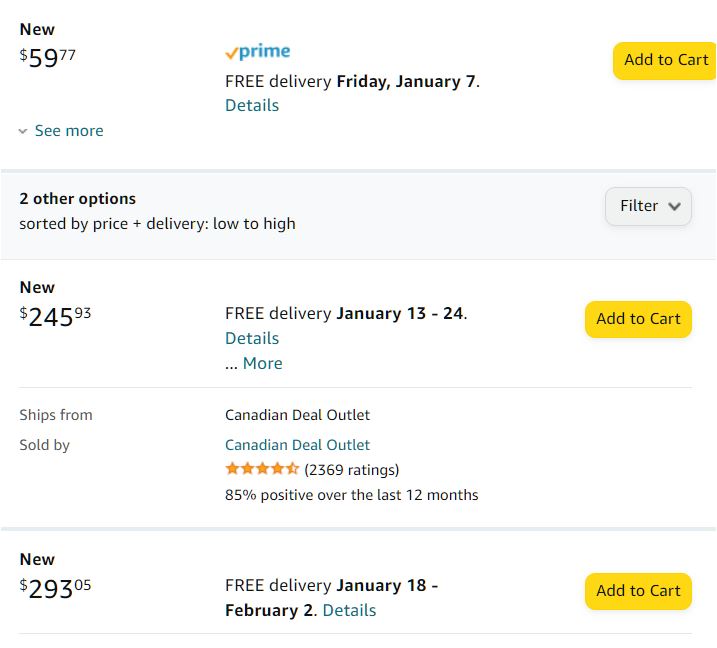This screenshot displays several product listings on Amazon Prime. At the top, the first listing indicates it is a "New" item priced at $59.77, available with Prime and includes free delivery by Friday, January 7th. Directly beneath this information, there is a "Details" button. Adjacent to it, there's a "See More" drop-down arrow, and to the right is a yellow "Add to Cart" button.

Below this, within a shaded light gray area, there is a note mentioning "Two other options," sorted by "Price + Signed Delivery, Low to High." Beside this, there is a filter button with a drop-down arrow.

The second listing is marked as "New" and priced at $245.93, with free delivery scheduled between January 13th and January 24th. Similar to the first listing, it features a "Details" link and a "More" link, with a yellow "Add to Cart" button on the right. Additionally, it specifies that the item ships from and is sold by "Canadian Deal Outlet." The product has a rating of 4.5 stars out of 5, based on 2,369 reviews, with 85% positive feedback within the last 12 months.

The final listing shown is marked as "New" with a price of $293.05, and it offers free delivery estimated between January 8th and February 2nd. As before, it includes a "Details" link and a yellow "Add to Cart" button on the right.